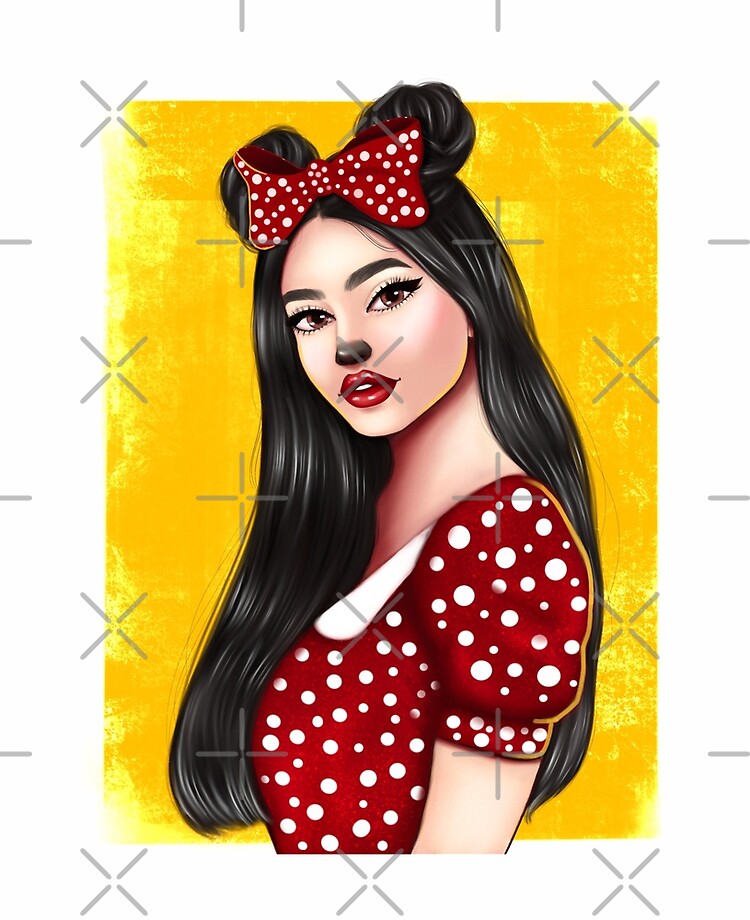This is a computer-generated image framed inside a white border with multiple decorative X's and lines, featuring a captivating young woman, possibly around 18 or 19 years old, in a detailed Minnie Mouse outfit. The main backdrop is a rustic, dark yellow rectangle resembling a playing card. The woman is presented in a profile stance, with her chest facing left and her back to the right, but her head is turned towards the viewer, giving a direct and engaging gaze with her striking hazel eyes. She has long, flowing black hair that extends down her back and front, styled into two buns on top of her head to mimic Minnie Mouse ears. A red bow with white polka dots sits prominently between the buns. Her expressive face is marked by thick black eyebrows, dramatic eye makeup, big lips with bright red lipstick, and a black-tipped nose to enhance the Minnie Mouse theme. She wears a short-sleeved red top adorned with white polka dots and a white collar. The attention to detail in her appearance, including her intricate hairstyle and vivid makeup, adds to the image’s striking and whimsical allure.